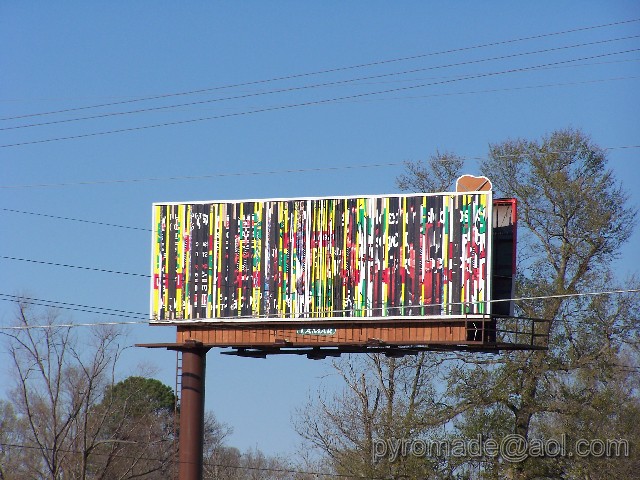A photograph captures a roadside scene featuring a large billboard. The backdrop reveals a clear blue sky dotted with power lines. In the distance, a line of trees provides natural contrast to the man-made elements. The billboard itself is elevated by a brown pole equipped with an attached ladder. Interestingly, the display on the billboard appears to be distorted. This could be a static billboard caught mid-transition between advertisements, revealing a mishmash of yellow, red, and brown colors alongside jumbled text. Another possibility is that it is an electronic billboard experiencing a malfunction. At the lower edge of the image, there is a visible watermark that reads "pyromade at aol.com," likely identifying the photographer.